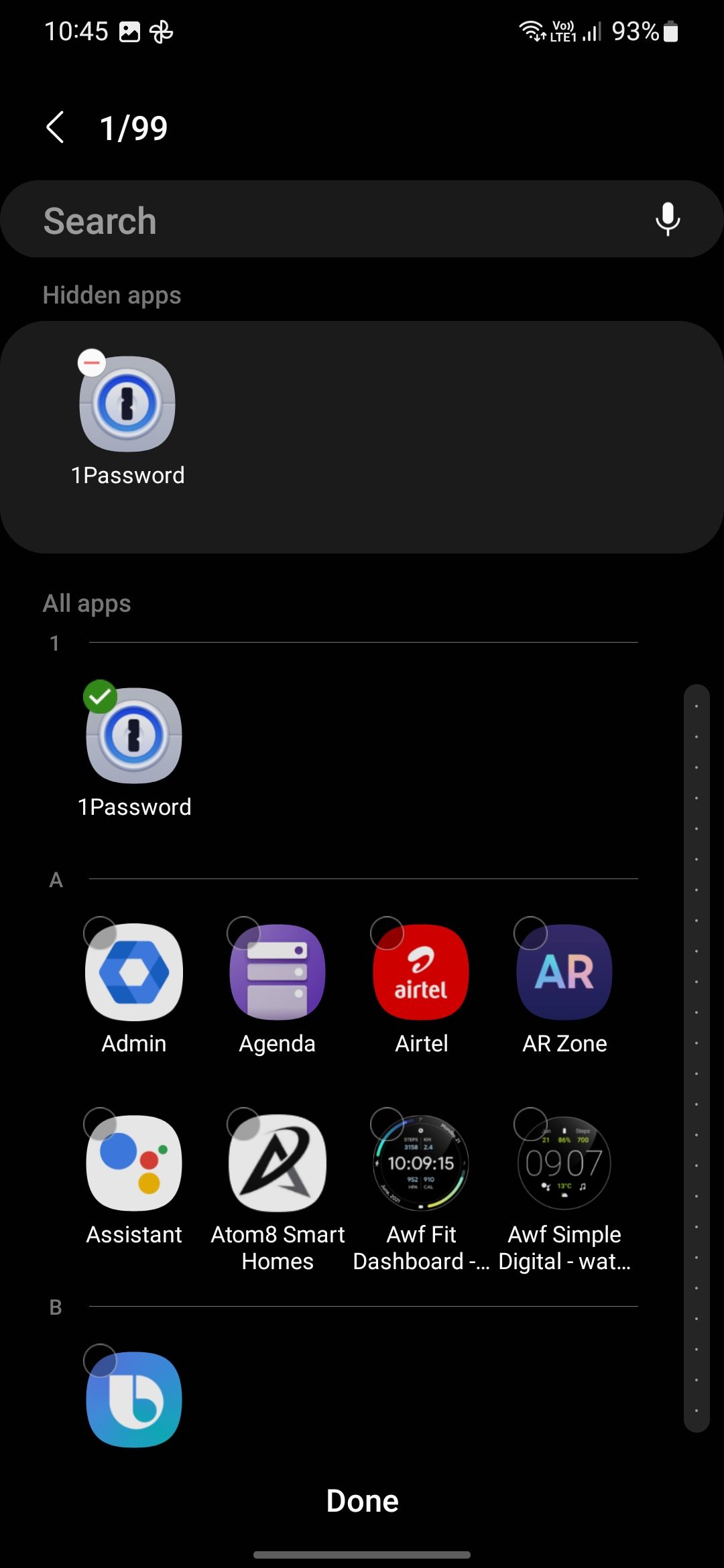The image appears to be a screenshot of a smartphone's home screen with a predominantly black and white theme. In the upper left corner, the background is black, transitioning to white within the display. The time is shown as "10:45", and to the right, a battery icon indicates a charge level of 93%. Below the time and battery, "1 of 99" is displayed, suggesting there are multiple screens or notifications. 

A search bar is prominently placed underneath these indicators. Following the search bar, there is a gray input field labeled "Password" with a distinct gray button below it, characterized by a black line through the middle and encircled by a blue border, likely an interactive element.

Further down, there is a black section labeled "All Apps." Beneath this section, there is a divider line followed by a grid of eight app icons arranged in two rows. From left to right, the apps in the first row are: "Admin," "Agenda," "Airtel," and "ARZone." In the second row, the apps listed are: "Assistant," "Atom 8 Smart Homes," "AWF Fit Dashboard," "AWF Simple Digital," and next to them, "WAT." 

At the bottom of the screen, within the "B" label category, there is an app with a blue icon featuring a white center that resembles the letter "B." Finally, at the very bottom of the screen, there is a "Done" button in black with white text, indicating the option to complete or exit the current task.